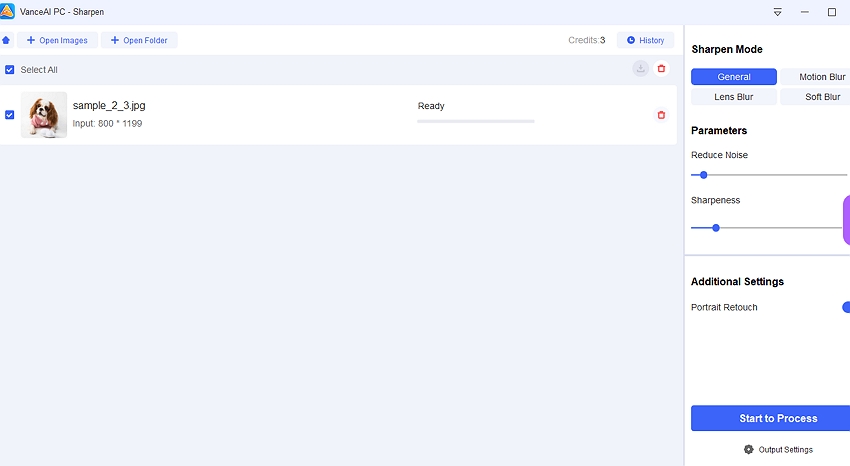The image features a user interface with a distinct light blue border at the top. In the top left corner, there is a logo consisting of a blue square with a gold object in the center and the text "Advanced AI PC-Sharpen" beside it. To the right, an arrow points downwards to a dash symbol and a square icon.

Below this, on the right side, there is a prominent labeled menu. At the top of the menu, it reads "Sharpen Mode." Directly underneath this title is a blue box labeled "General." Following it, there are three gray boxes labeled "Lens Blur," "Motion Blur," and "Soft Blur," respectively.

Under these options, there is a section labeled "Reduce Noise" accompanied by an adjustable bar, which is positioned almost all the way to the left. Below this section, another labeled "Sharpness" also features an adjustable bar, similarly positioned nearly to the left. Each adjustable bar is marked at both ends by blue circles.